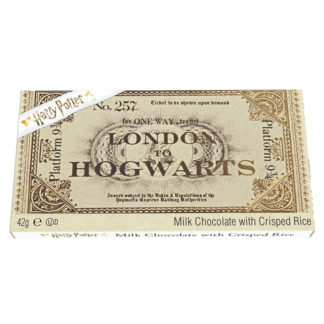This close-up image depicts a single chocolate bar still encased in an ornate wrapper designed to resemble a vintage train ticket. The beige-tan paper mimics a newspaper look, adorned with an intricate bronze-gold gear pattern that hints at British heritage. Dominating the top left corner is a white ribbon emblazoned with the familiar gold "Harry Potter" text. The wrapper prominently displays "Number 257 for one way from London to Hogwarts" and "Platform 9 3/4," evoking a sense of magical journey from the Harry Potter series. The lower right-hand corner identifies the treat as "milk chocolate with crisp rice," weighted 42 grams. The chocolate bar is centered against a stark white backdrop, suggesting a stock image setting, likely used for online candy shopping.